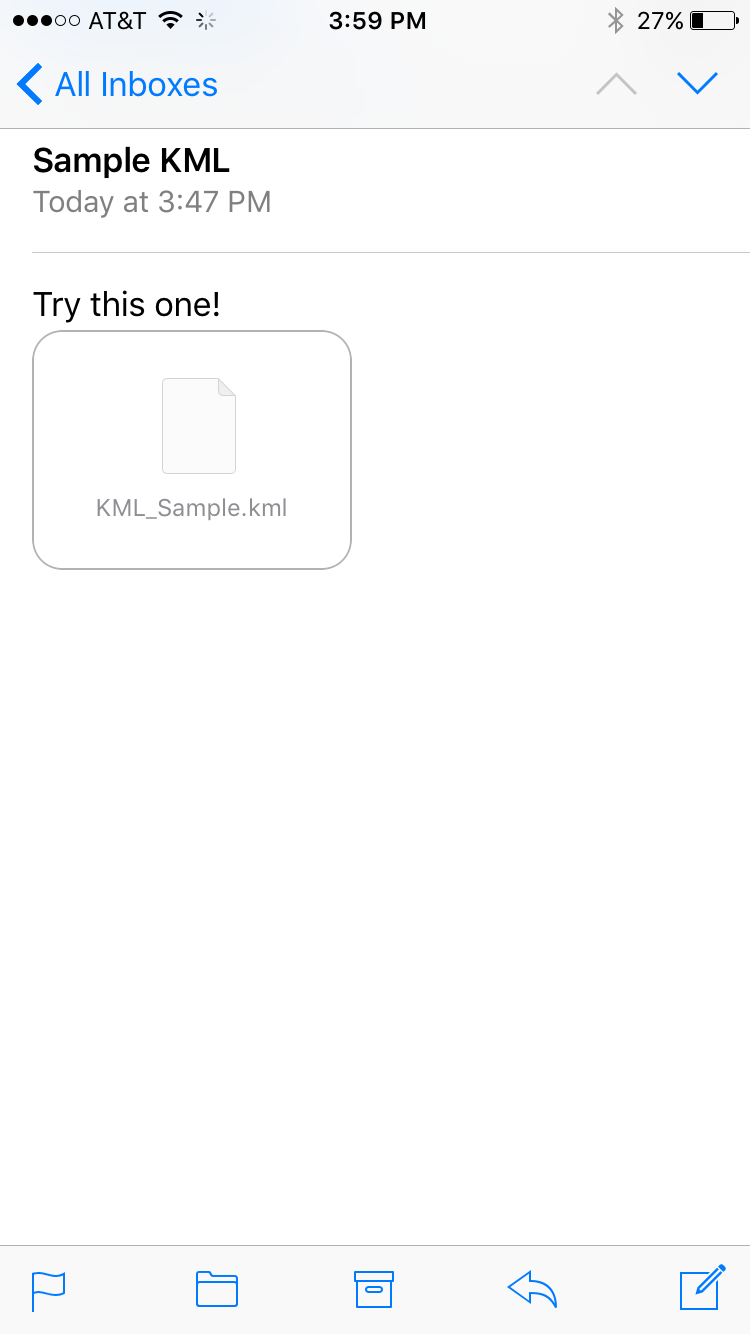This is a detailed screenshot of a phone displaying the Gmail app. At the top, there's a grey status bar showcasing various icons. On the left, signal strength is depicted with five dots, three of which are black and two are white in the middle. This is followed by the "AT&T" label, the Wi-Fi symbol, and a loading icon. The time is shown as 3:59 p.m. on the right side of the status bar. To the far right, there’s a Bluetooth icon, the battery level at 27%, and an accompanying battery symbol. Below the status bar, blue up and down arrows are visible, with the down arrow colored blue and the up arrow grey. 

On the left, the label "All inboxes" is highlighted in blue with a left-pointing arrow next to it. Beneath this, the email's subject "Sample KML" is displayed in bold black letters. The timestamp "Today at 3:47 p.m." appears in smaller, grey font underneath the subject line. The email body is succinct, containing the text "Try this one!" followed by an attachment icon and the file name "KML_sample.KML."

At the bottom of the screen are several functional icons: a flag, a folder, a box, a share arrow, and a button for composing a new message.